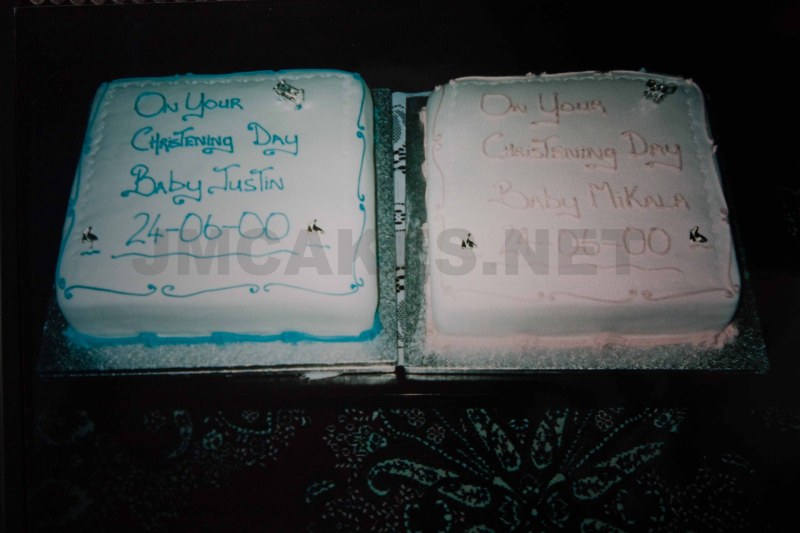This is a watermarked photograph from jmcakes.net featuring two white christening cakes for twin babies, Justin and Mikala, taken on 24-06-00. Each square cake sits on a slightly larger aluminum base and is set against a very dark background. The cakes are nearly identical except for the color schemes: one has blue piping and lettering for baby Justin, reading "On your christening day, baby Justin 24-06-00" with elaborate scrolling, while the other is adorned with pink piping and lettering for baby Mikala, spelling out "On your christening day, baby Mikala 24-06-00." Both cakes have piped borders in their respective colors accentuating their bases.